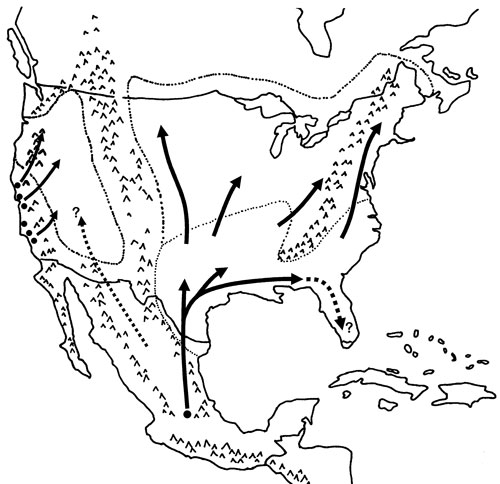This is a detailed black and white drawing of a map encompassing the United States and parts of Canada, Central America, and the Caribbean, including Cuba and islands near Florida. The map, which lacks any labels or wording, features a network of arrows possibly representing weather patterns, wind currents, or migration flows. These arrows originate from the Pacific Ocean, traversing through Latin America and dispersing in various directions across the United States, toward New England, and reaching up to the Canadian border. The map also contains inverted V shapes indicating mountain ranges. Despite the ambiguity of what exactly the arrows denote—whether weather phenomenon or migration pathways—the visual intricacy and directional flow patterns are prominently illustrated.